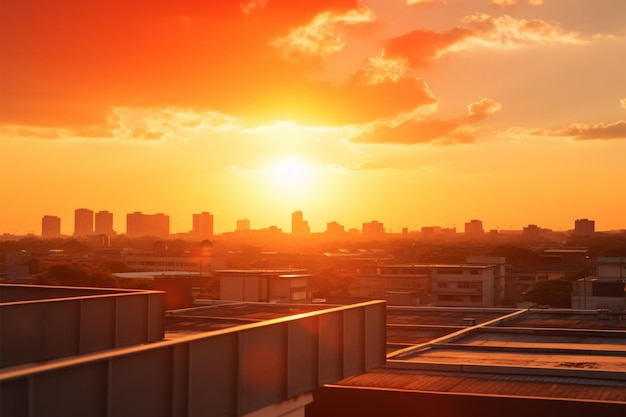This is a wide-angled landscape photograph capturing the vibrant scene of a city as the sun nears sunset. The sky is ablaze with hues of bright orange, dark red, and yellow, reflecting off thick clouds that add texture to the backdrop. The silhouette of the city skyline is visible in the distance, with multiple high-rise buildings reaching upward. Closer to the foreground, a mix of commercial and residential buildings with flat, metal rooftops dominate the view. The entire scene is bathed in a warm, amber glow, suggesting the heat of the day. The angle of the sun casts long shadows and highlights the reflective surfaces of the buildings, creating a striking interplay of light and color. This detailed image portrays a serene yet dynamic urban landscape at the golden hour, symbolizing the transition from day to night.